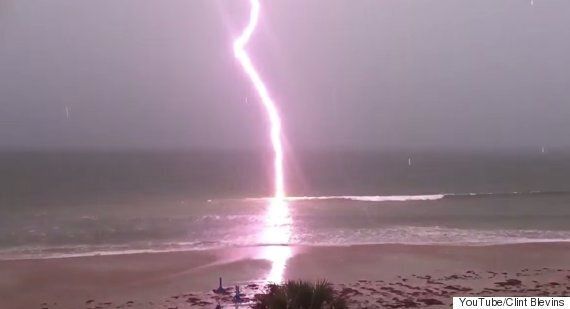The photograph captures a striking scene of a powerful lightning bolt hitting the ocean amidst a tumultuous storm. The foreground showcases wet, tan-colored sand, and at the very center bottom, a tuft of green vegetation, possibly grass, stands resiliently. The ocean itself appears dark gray, except where it is dramatically illuminated by a vibrant lightning bolt that features a stunning pinkish-purple hue. This bolt cuts through the sky from the top center down to the mid-center of the image, striking directly in the water, which is frothing white as waves crash against the shore. The sky above mirrors the ocean's mood with its dark gray, storm-laden clouds, contributing to the overall murky yet awe-inspiring atmosphere of the photograph.